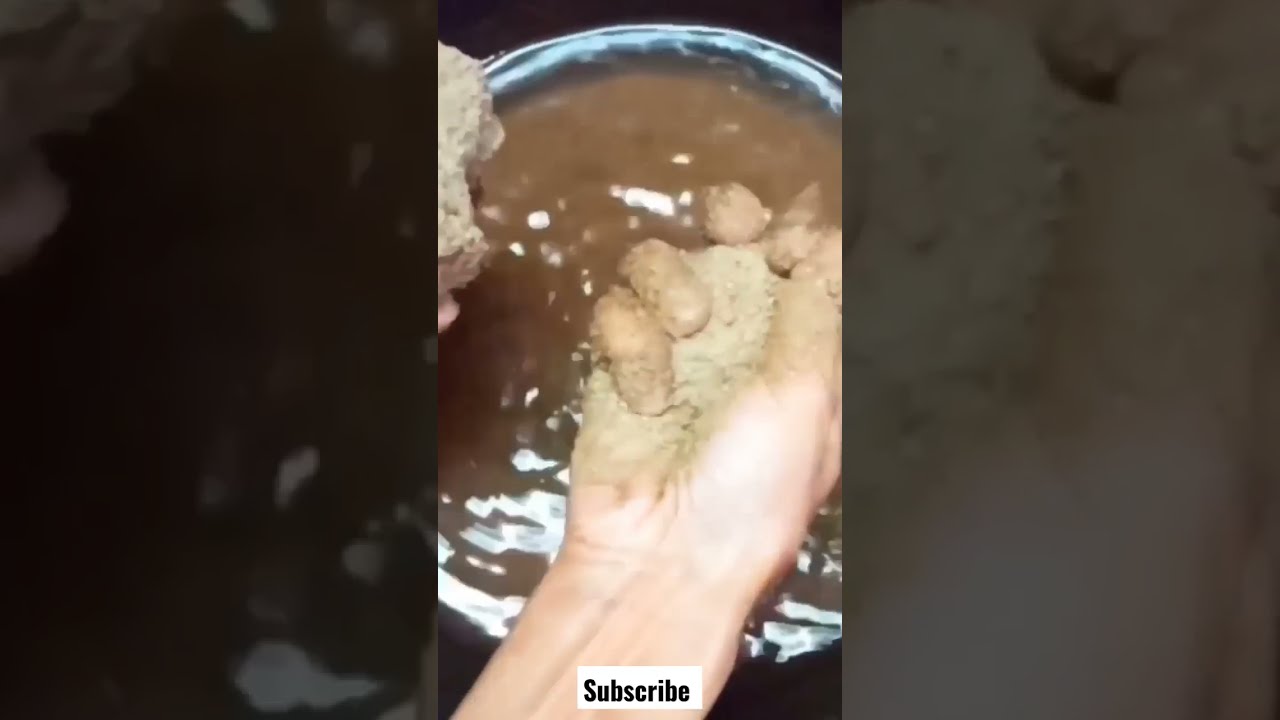This image, viewed from above, features a pair of hands over a glass bowl containing a gelatinous, muddy brown substance. Positioned in the center, the right hand is clearly visible from the lower forearm to the fingers, which are clasping a light brown, powdery material. The partially visible left hand shows only the tops of fingers, also dusted with the same brown powder. The backdrop of the image consists of two equal-sized rectangles on either side, each darkened and blurred. The one on the left shows a close-up of the muddy water in the bowl, and the one on the right displays an enlarged view of the hand holding the brown substance. Overlaying the bottom center of the image, in a white rectangle with black lettering, is the word "subscribe," indicating it's a promotional image likely sourced from an online channel.